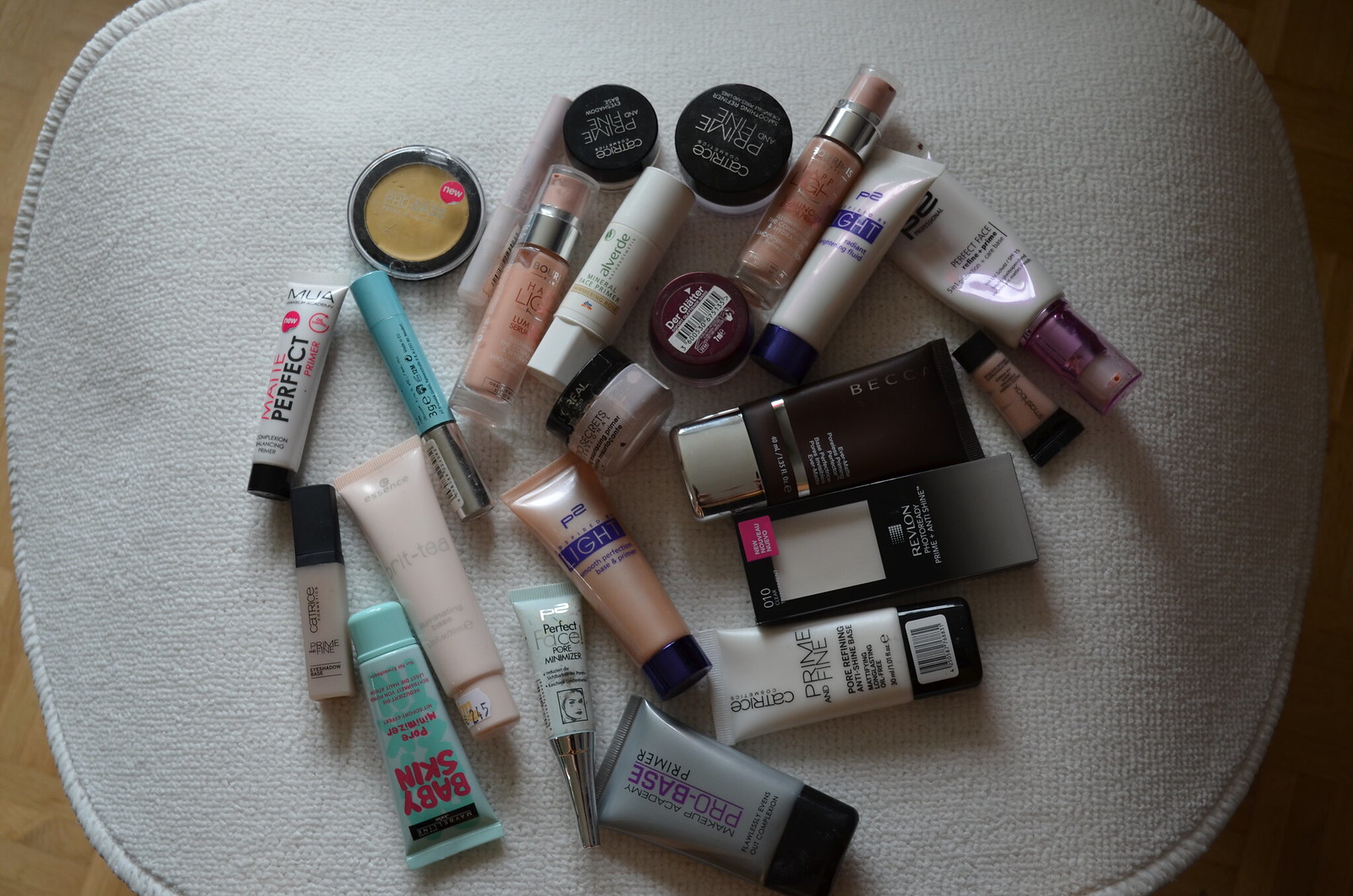In this captivating bird's-eye view photograph, a rectangular, landscape-oriented image showcases a meticulously arranged array of makeup products spread out on a pristine white cloth, which itself rests elegantly on a tabletop. The white cloth, circular in shape, features a finely-knit trim around its edges, adding a touch of sophistication to the display.

A plethora of makeup items—approximately 23 in total—are artfully placed, creating a visually appealing assortment. Among these, five circular containers stand out, typically housing lip gloss or bronzer. On the left, one such container is transparent, revealing a light bronze shade within. This container bears the label "Red New" encircled in text.

At the top, two prominently branded items are easily identifiable. One is labeled "CATRICE Prime Fine," while the other below it reads "DERGLATTER" with a scanning code underneath. Another cylindrical item rests on its side with the word "Secrets" clearly visible.

Multiple tubes and containers of various shapes and sizes fill the remaining space. Notably, there is an open box prominently displaying the brand "Revlon." Most items are positioned upright, making their labels readable. Among these labels are phrases such as "Prime Fine," "Pro Base Primer," "Baby Skin Perfect Pore Minimizer," and "Light Matte Perfect Primer," indicating that these products primarily consist of face foundations, bronzers, and primers, intended to enhance and alter the complexion rather than lip products.